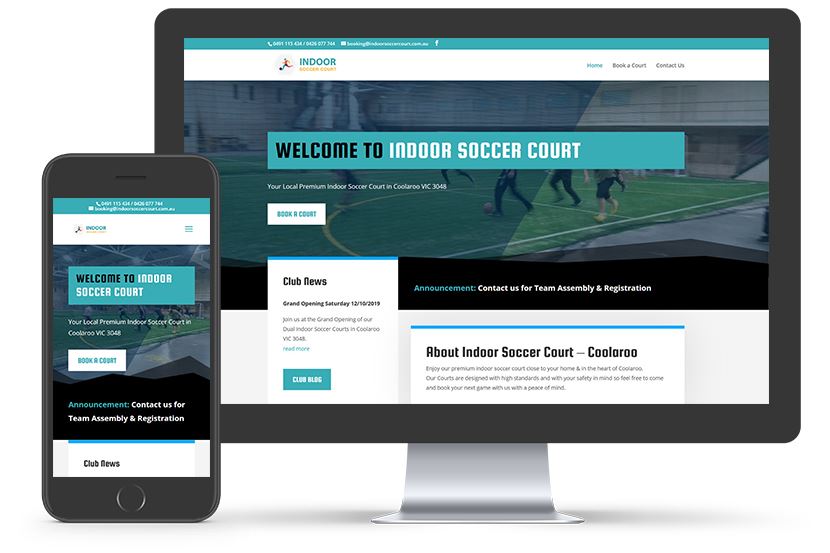This image showcases a mock-up or advertisement for an indoor soccer court website, displayed on both a desktop computer and a smartphone. The background is white, blending seamlessly into the environment. Centrally, there's an image of what appears to be a desktop Mac computer, evidenced by its silver stand and distinctive shape, although the Mac icon is not visible. The computer screen features the website, which utilizes a color scheme of teal, white, and black.

Below and in front of the computer screen, positioned on the lower left corner, is a black smartphone standing up. The phone also displays the same website, but adapted to fit the smaller screen with appropriate spacing and formatting changes. Both the desktop and mobile versions prominently feature the message "Welcome to Indoor Soccer Court" with "Welcome to" in black text within a teal box, and "Indoor Soccer Court" in white text. The presence of the same visual elements on both devices indicates the website's responsive design, highlighting its adaptability across different platforms.